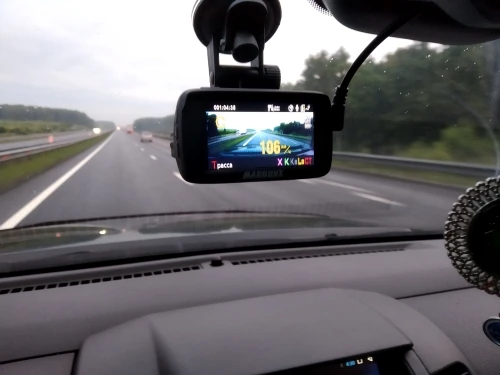The photo, taken from the driver's seat inside a car with a gray interior, captures a view of a dull, cloudy day on a highway. The car is traveling in the left lane of a divided, two-lane highway, marked by a dashed white line separating it from the adjacent lane. The heads-up display shows a speed of 106 kilometers per hour. The highway is bordered by guardrails on both sides, with more trees and greenery on the right side and mostly grass on the left. In the distance, a couple of cars are visible in the right lane. Additionally, there are headlights from vehicles on the opposite side of the grass median. Inside the car, part of a small fan is visible on the dashboard to the right, and atop the dark gray dashboard surface, a black monitor is attached to the windshield, displaying a digital, zoomed-in view of the road ahead.